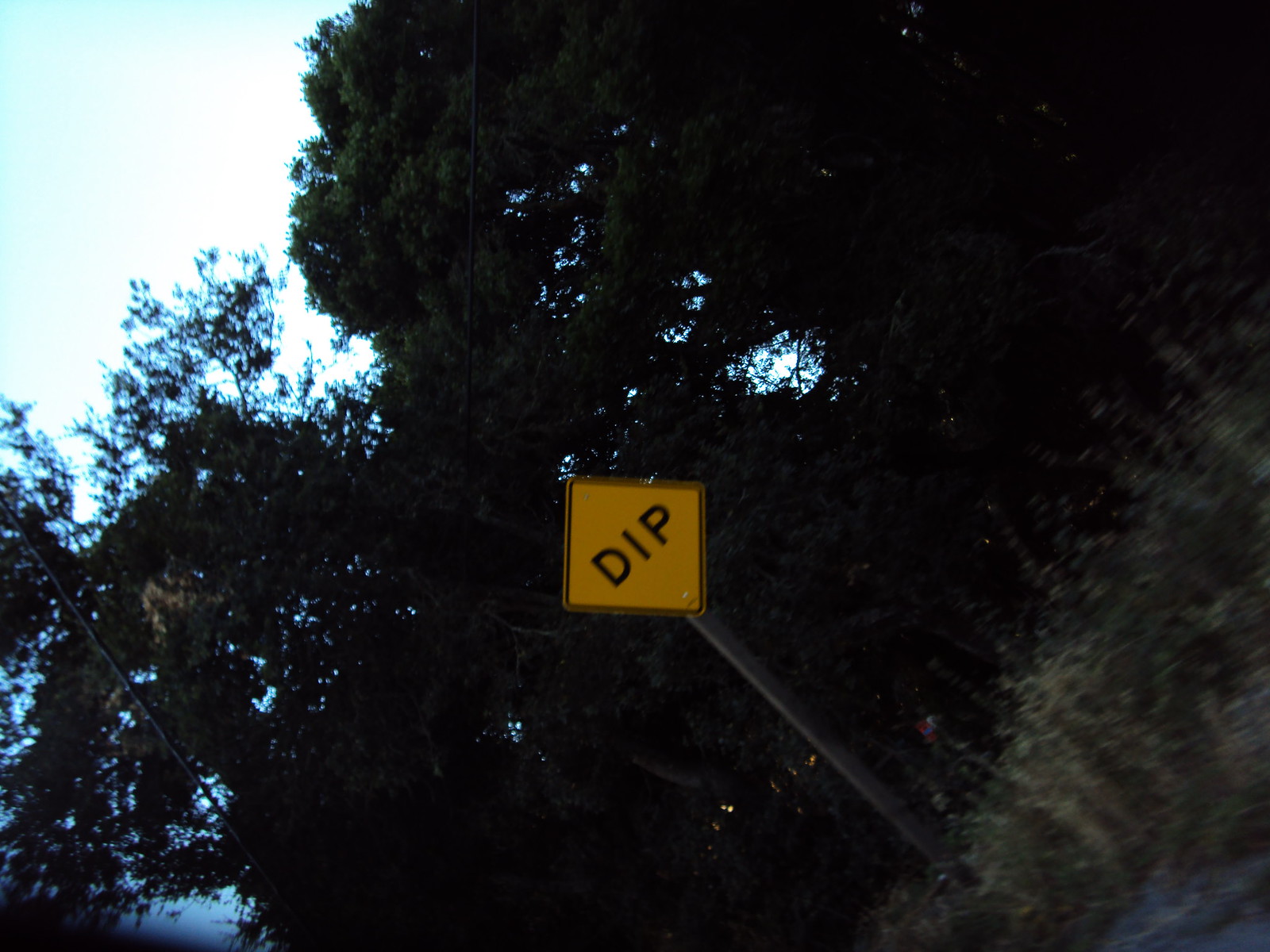The photographic image captures a dark, densely wooded area, giving an impression of peering through thick, black silhouetted foliage. The scene is shrouded in dim lighting, with no apparent sunshine and an absence of color. To the left, a patch of sky appears overexposed, exhibiting a washed-out white-grey hue. In the middle of the composition, a small, square, orange road sign stands out against the dark backdrop. The sign, with large black letters, reads "DIP," suggesting a warning for an upcoming dip in the road. The precise setting is ambiguous, possibly a deep forest, a wooded area, or even a tree-lined avenue. The overall mood is mysterious and somber, with limited visibility and an obscure atmosphere.